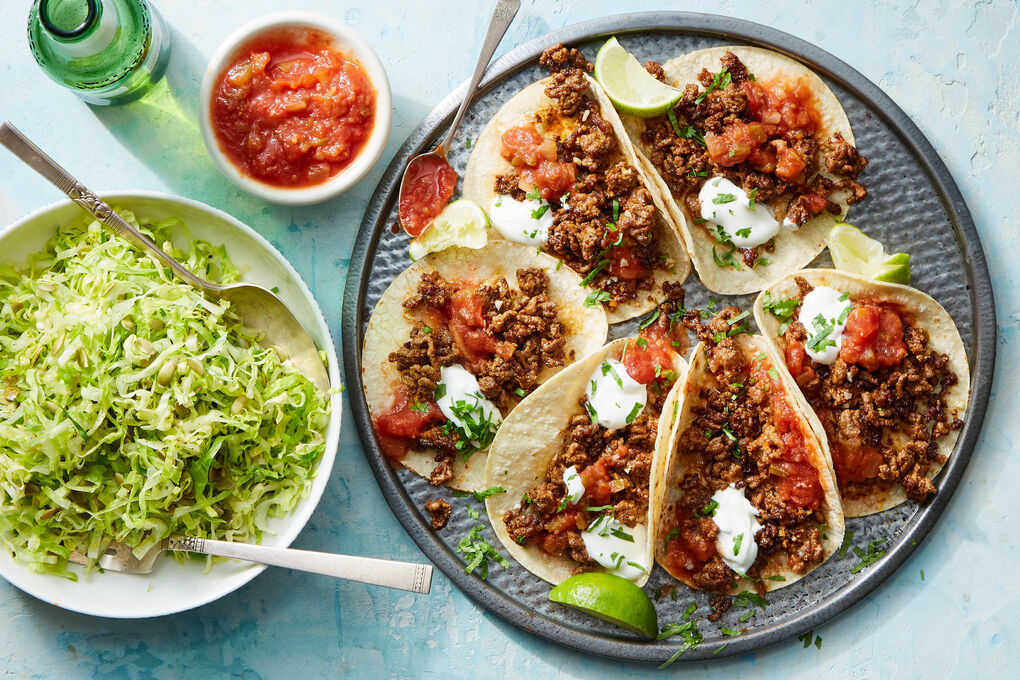This photograph captures a meticulously arranged dinner setting on a light blue concrete surface, viewed from above. Central to the image, a large, dark gray circular metal dish holds six generously filled soft tacos. Each taco is packed with browned meat, fresh chopped tomatoes, sour cream, and a sprinkling of chives and cilantro. A silver spoon for serving is placed beside the tacos on the pan. To the right of the taco dish, a large white bowl brimming with shredded green lettuce is accompanied by a silver fork and spoon. Above and slightly between the two main dishes, a small white porcelain bowl contains vibrant salsa. In the upper left corner, the top of a green glass bottle, possibly soda or beer, peeks into the frame, adding a touch of casual beverage presence. Lime wedges scattered around enhance the festive, appetizing appearance of the meal.